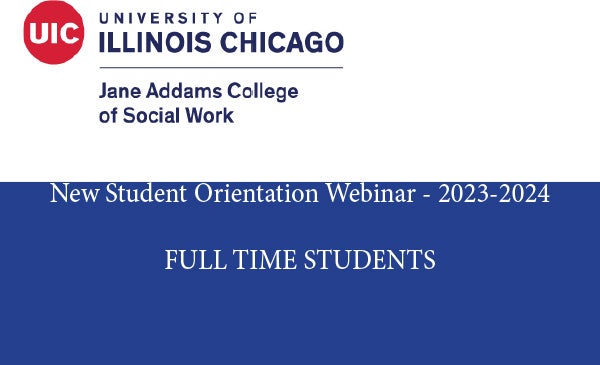This image is a screenshot featuring the branding and information from the University of Illinois Chicago (UIC). At the top left corner of the image, there is a distinctive red ball with the white letters "UIC" inside it. Adjacent to the red ball, in small blue text, is the phrase "University of", followed by "Illinois Chicago" in significantly larger blue text, approximately 60-point font. 

Beneath this, there is a thin blue line, under which the text "Jane Addams College of Social Work" is written in an 18-point font, spanning two lines.

The upper half of the image has a white background, while the lower half is dominated by a blue rectangular box. Inside this blue box, in white font at the top, the text reads "New Student Orientation Webinar – 2023 – 2024". Midway down the blue section, it states "Full-Time Students" with some space separating it from the aforementioned orientation text.

All text in the top white section is aligned to the left corner of the image. Notably, the blue used in both the "University of Illinois Chicago" text and the blue box at the bottom appears to be identical, creating a cohesive color scheme. The white text remains consistent throughout the image, ensuring clear visibility and uniformity.